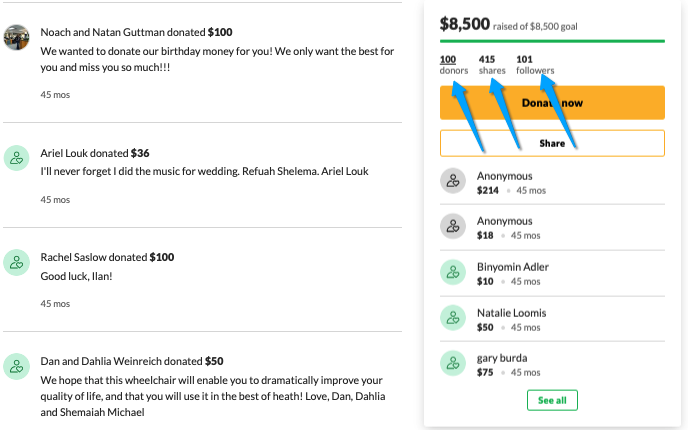**Detailed Descriptive Caption:**

This image is a screenshot of a fundraising webpage with a predominantly white background. In the top left-hand corner, there are four sections delineated by thin gray lines. At the very top section, there is a circular profile picture of an individual or user. To the right of this image, composed in a gray uppercase and lowercase font, it reads: "Noach Natan Guttman donated $100." Following this, the text in smaller font expresses their heartfelt message: "We wanted to donate our birthday money for you! We only want the best for you and miss you so much!!!" Below this message, in a smaller gray font, it states "45 MOS" indicating that the donation was made 45 months ago.

The next section has a teal background featuring the silhouette of a person with a head, torso, and a heart. Within this section are the details of Ariel Louk's contribution. It says, "Ariel Louk donated $36" followed by her message: "I'll never forget I did the music for your wedding. Refua Shalema Ariel Louk."

The third section is about Rachel Saslow's donation: "Rachel Saslow donated $100," accompanied by a brief note: "Good luck Lian!" Once again, it states "45 MOS" indicating the time of donation.

The final section details the donation from Dan and Dahlia Weinreich: "Dan and Dahlia Weinreich donated $50." Their message reads: "We hope that this wheelchair will enable you to dramatically improve your quality of life, and that you use it in the best health! Love, Dan, Dahlia, and Shemaiah Michael."

In the top right-hand corner of the image, separated by a vertical line, there is a summary of the fundraiser's progress. A dollar symbol indicates $8,500 raised of the $8,500 goal. Below this is a thin green line, with three long blue arrows pointing to the below metrics: "100 donors," "415 shares," and "101 followers."

At the bottom of the screenshot, there is a large yellow button labeled "Donate Now" in black font. Adjacent to this button is another outlined in yellow, with the word "Share" in black. Below these are further details showing contributions by anonymous donors.

The entire layout of this image clearly highlights the contributors and their messages, as well as the progress and call-to-action buttons for the fundraising campaign.